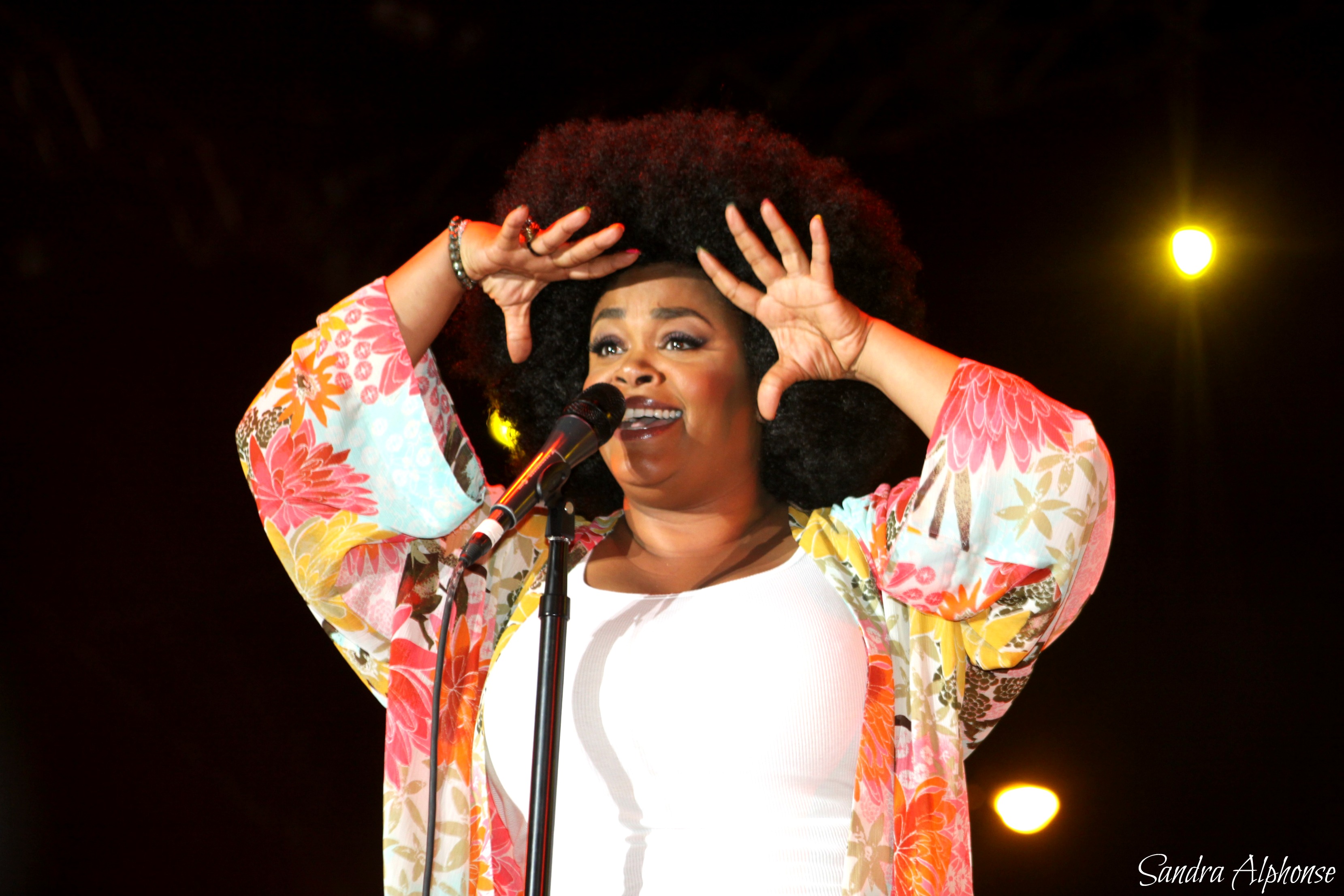In this photograph, we see an African American woman, likely aged between 30 and 35, standing confidently as she sings into a black, wired microphone. She has a large, thick, fluffy afro and wears dark red or dark brown lipstick along with eyeliner, accentuating her expressive, bright eyes and joyful smile. She is dressed in a well-fitted white tank top or short-sleeve shirt, layered with a vibrant floral-patterned long sleeve shirt or jacket. The woman is captured with both of her hands raised near her face, as if she's shading her eyes to look for someone in the audience, adding an element of expressiveness to her performance. The background is pitch black, punctuated only by two light sources—a yellowish one near the right side and a small, orangish one at the bottom right. In the lower right-hand corner, in white cursive font, the name "Sandra Alphonse" is displayed, suggesting either the photographer or the performer's name. The photograph, which is horizontally aligned in a rectangle shape, beautifully captures this moment of vibrant auditory expression and visual delight.